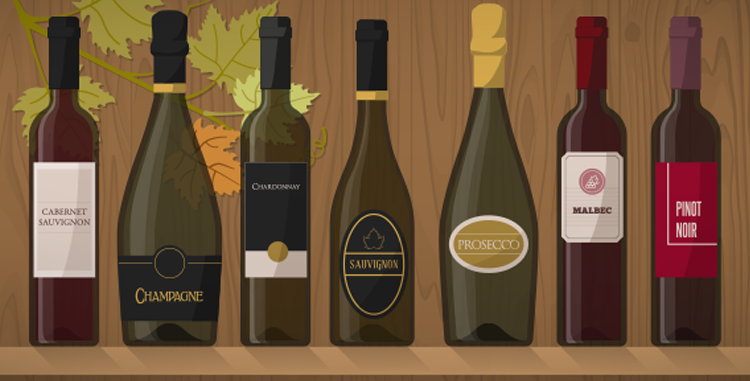This illustration features a cartoon-style depiction of seven wine bottles arranged on a light brown wooden shelf, set against a medium brown wooden wall distinguished by prominent vertical grains. From left to right, the bottles, varied in color and label, nearly span the height of the entire image. At the upper left corner, a greenish branch with three light green leaves and one orange leaf extends into the scene, adding a touch of nature.

The first bottle, with a black wax seal and a white rectangular label, is a Cabernet Sauvignon. The second bottle, a dark green Champagne bottle with a black label inscribed in muted yellow, also features a black wax seal. Next is a green Chardonnay bottle, labeled in white on a black rectangular label, again topped with a black seal.

The fourth, another dark green bottle, is marked Sauvignon with gold lettering on a black, oval label with gold trim, and likewise has a black top. Beside it, the fifth is a Prosecco bottle, its label golden with white trim, topped with a light yellowish-gold cap.

The sixth, a Malbec, closely resembles the Cabernet Sauvignon bottle but has a red wax top and a white label. Finally, the seventh bottle, a dark purple Pinot Noir, bears a brighter red label with white lettering and is capped with a muted purple seal.

Together, these bottles form a cohesive yet diverse collection, enriched by the meticulously illustrated wooden backdrop and leafy accent, capturing a vibrant and detailed tableau.